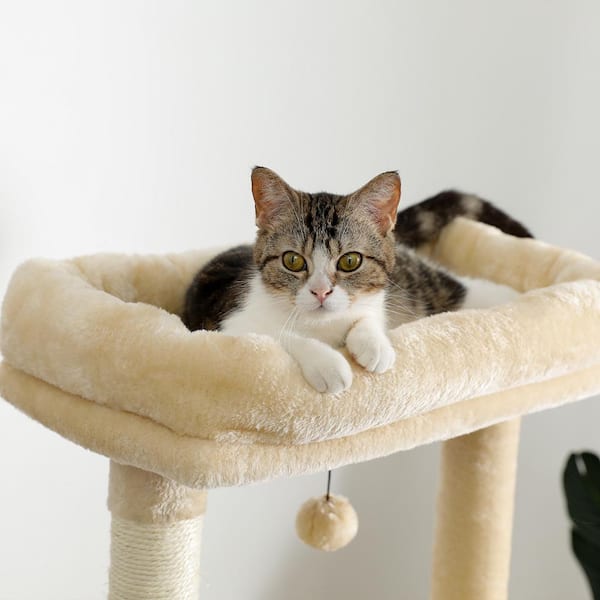The image features a domestic tabby kitten with distinct white paws, a white stripe on its face, and hazel eyes. The kitten is comfortably settled in a soft, furry basket-like bed. The bed features a white interior with cream-colored, fur-covered edges and is elevated on posts wrapped in twine. A cream-colored, fuzzy pom-pom hangs from the bed structure. The kitten's ears are perked up, and it gazes directly at the camera, with its two front paws draped over the edge of the basket. The background is a very light gray, and a small, black object is visible at the bottom right corner of the image.